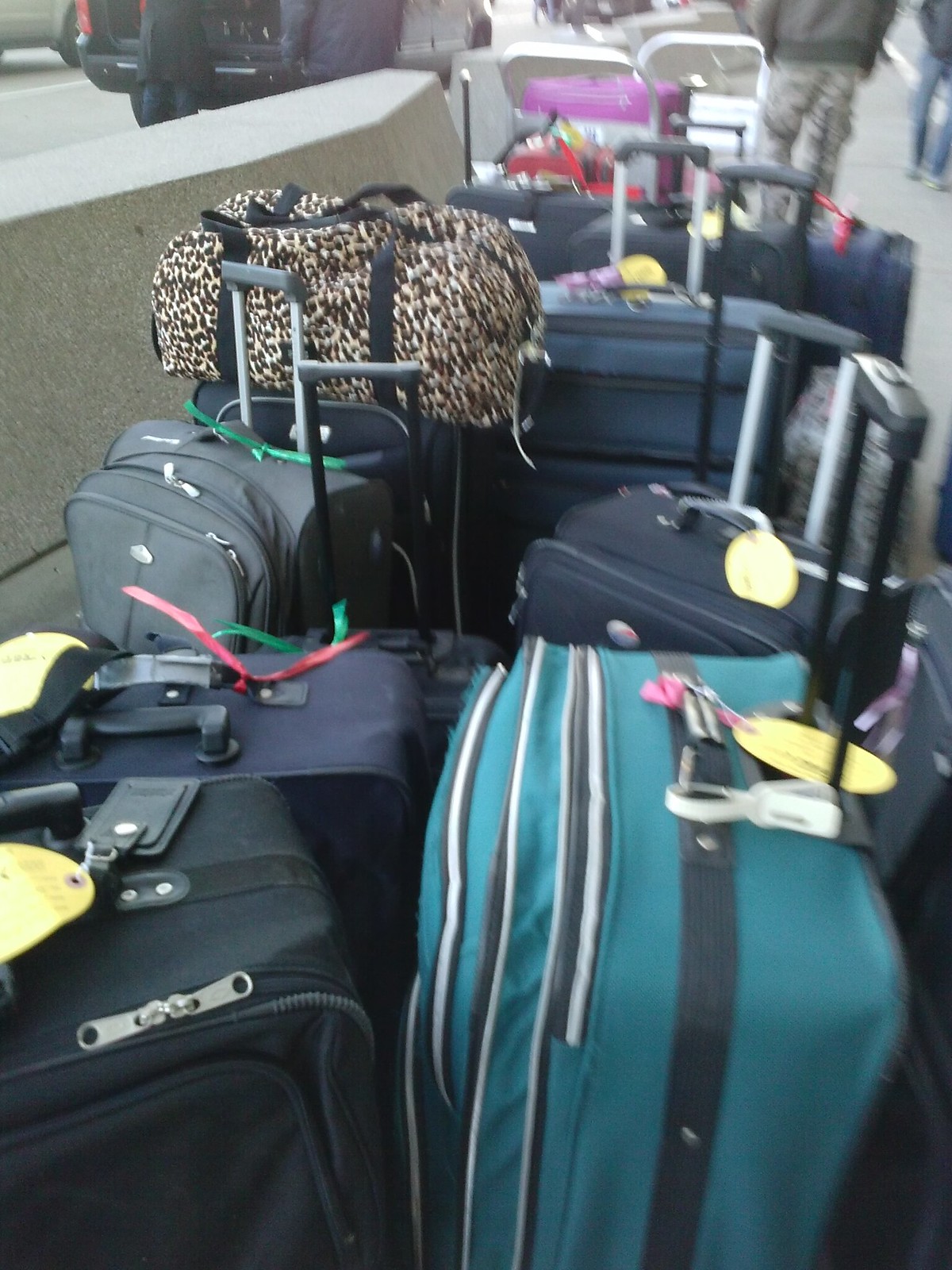This photograph captures a cluster of approximately eleven suitcases lined up on what appears to be a curb, likely outside an airport. The quality of the image is somewhat blurry, impacting both the background and foreground details. In the upper left-hand corner, part of a vehicle can be seen, likely in the process of unloading more luggage, accompanied by at least two people visible in the upper right-hand corner.

The suitcases are arranged with their handles mostly extended and come in a variety of colors. Predominantly, the luggage is black or dark blue, but notable exceptions add splashes of color and pattern. In the forefront, a teal-colored suitcase, along with several blue ones, each marked with yellow tags, is distinctly visible. A standout in the collection is a leopard-patterned bag perched atop a gray suitcase in the center. Further into the cluster, there are additional black, gray, and blue suitcases, with some appearing slightly faded due to the blurriness of the image.